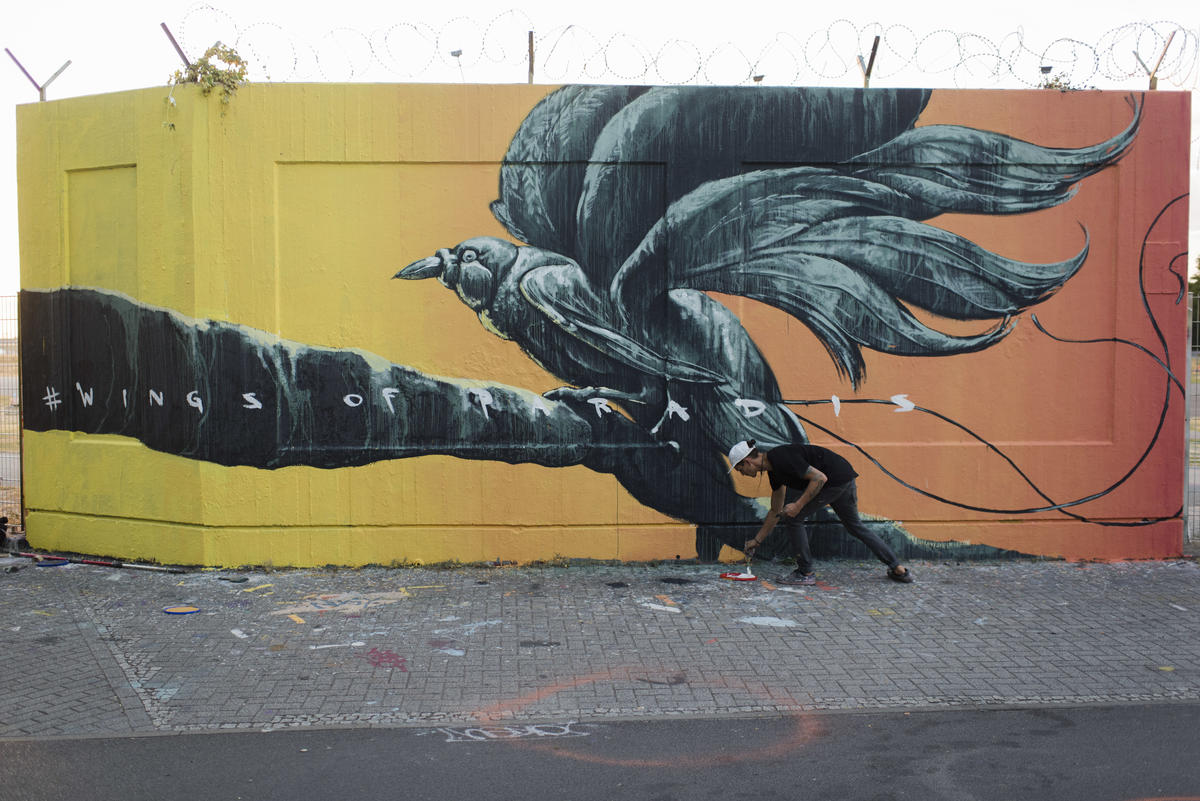The photograph depicts a young artist engrossed in painting a detailed street art mural on the side of a building. The image is in color and in landscape orientation, with an overcast sky casting a neutral light. The wall dominating the background angles near the side and stretches horizontally across the width of the image. At the top of the wall are metal bars adorned with spirals of barbed wire, indicating the building's urban setting. 

The vibrant mural features a surrealistic black bird, with outstretched wings that extend dramatically behind it, perched on a large black tree limb. Notably, the bird's beak is depicted as an ink pen tip, adding a touch of artistic symbolism. Surrounding the bird, the wall exhibits a gradient of colors, transitioning from yellow on the left to peach on the right. The words "#WingsOfParadise" are handwritten in white along the tree branch; however, the artist is in the process of finishing this text, as the final 'E' in "Paradise" has yet to be completed.

In the foreground, the young male artist, dressed in a white cap, black t-shirt, and dark jeans, is bent over, mixing white paint on a saucer placed on the cobblestone sidewalk. There are spots of paint scattered around him, evidence of his ongoing work. The mural, rendered in photographic representational realism, serves as both a striking visual and an expression of creativity against the rugged and fenced urban landscape visible on either side of the wall.